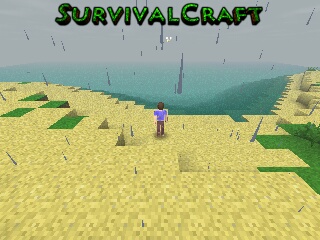The image depicts a video game screen titled "Survival Craft" in large green letters, with slightly larger 'S' and 'C'. All letters are capitalized. Dark raindrops fall over a scene featuring a blocky, human-like figure reminiscent of Minecraft, wearing a blue shirt and brown pants, with brown hair. The figure stands on a yellow surface with green patches, suggesting a grassy terrain. In the distance, there is a greenish-blue area, indicative of water. The entire scene is rendered in a distinctly blocky, pixelated style, typical of Minecraft-inspired games.